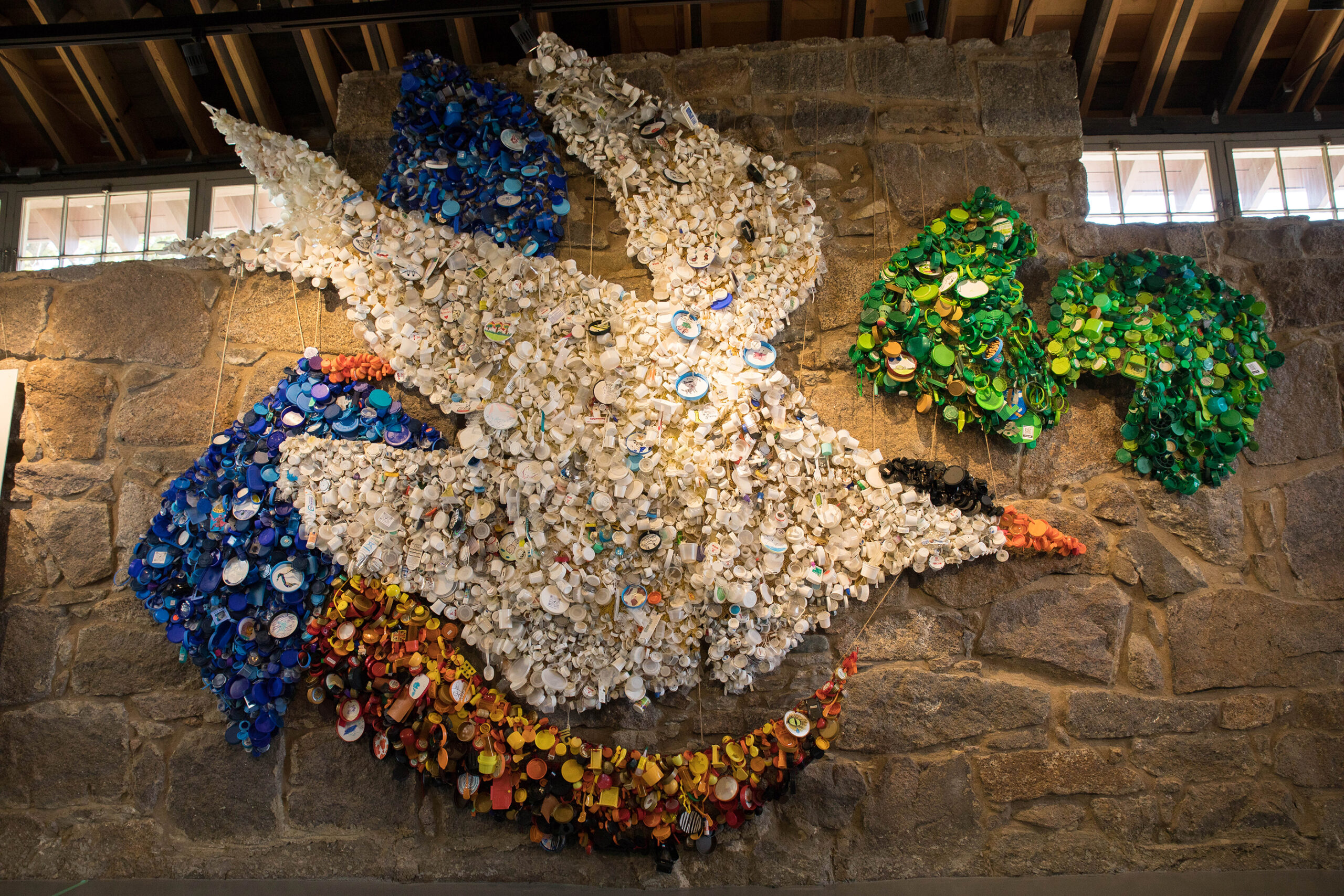The photograph captures a large indoor brick wall adorned with a striking mosaic artwork. The wall features narrow windows, possibly barred, situated at the top left and right corners. Above, an industrial roof constructed with metal and wood beams spans the length of the image. Central to the composition is an intricate mosaic, crafted from materials that appear to be seashells, sea glass, or recycled items, creating a vivid and textured effect. The mosaic depicts a bird, likely a seagull, with a bright orange beak, a black-domed head, and wings seemingly in flight amidst swirling hues of bright blue and white. Below the seagull, an orange shape resembling a dinosaur's tail or a curved arc adds a dynamic element, hinting perhaps at clouds. To the upper right of the bird's head, green shapes resembling treetops contribute to the rich, layered scene, all illuminated by subtle spotlighting that enhances the colors and textures of the artwork.